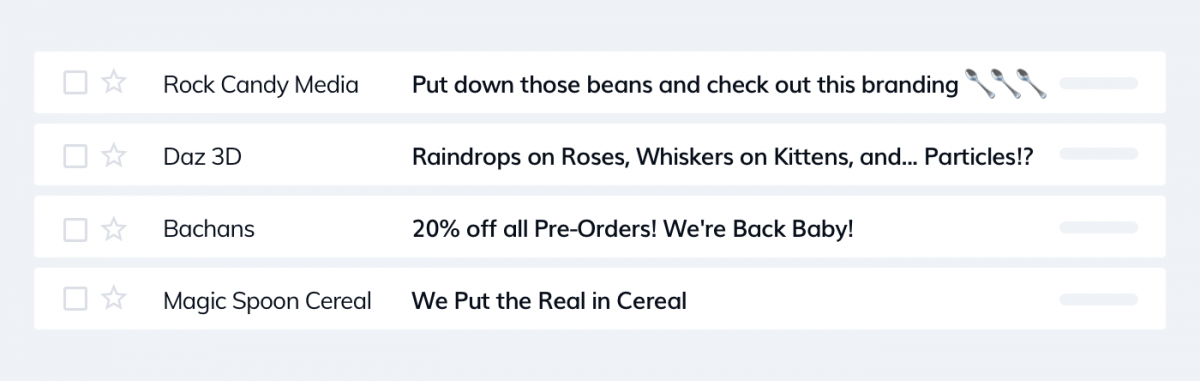The image appears to be a partial screenshot of a webpage, mainly featuring a large light gray rectangle divided into four smaller sections, each containing checkmarks, stars, and various texts. 

1. The first section contains a checkmark and a star, with the text "Rock Candy Media." Below this, it reads, "Put down those beans and check out this branding," accompanied by three spoon emojis.

2. The second section also features a checkmark and a star, and is titled "Dad's 3D." The accompanying text states, "Raindrops on roses, whiskers on kittens, and... particles?" with the dot-dot-dot implying confusion.

3. The third section includes a checkmark and a star, with the headline "Batchons." The text highlights a promotion: "20% off all pre-orders. We're back, baby!"

4. The final section again showcases a checkmark and a star, and is labeled "Magic Spoon Cereal." The text reads, "We put the real in cereal."

Each section offers the ability to interact with the checkmarks and stars, likely indicating areas for user ratings or selections. The overall color scheme of the image consists of white, light gray, and black tones. This screenshot captures a segment of a website, emphasizing its branding, promotional offers, and interactive elements.